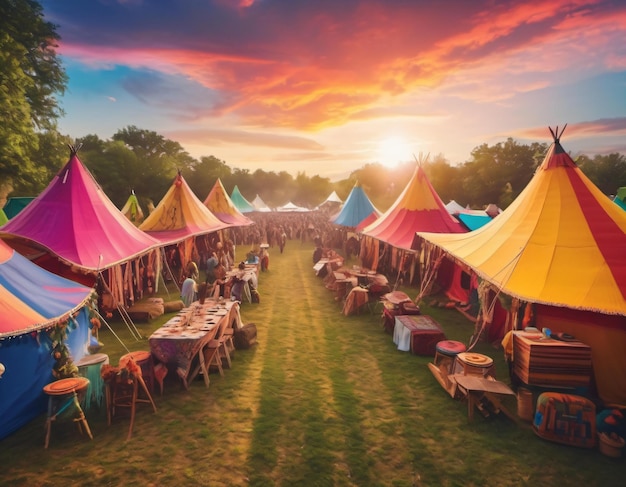This painting depicts a vibrant street fair or market scene under a beautiful twilight sky. The sky transitions from blue to shades of pink and yellow, with clouds adding depth to the scene. The fairground is framed by trees that provide a natural border, with tents lining both sides of a grassy central lane that extends into the distance. The tents are various cheerful colors including yellow, turquoise, pink, blue, and red, each sheltering tables, stools, and a blur of indistinct figures suggesting a bustling crowd. On the left, a blue tent occupies the bottom corner, followed by a pink tent with tables and chairs in front, extending to more tents and tables with people behind them. On the right side, a yellow and red tent stands out, with boxes stacked in front and small wooden tables nearby. Additional colorful tents and tables continue down the grassy path, guiding the viewer's eye towards a white tent far off in the distance. The horizon line is punctuated by a tree on the upper left, and more tents extending across the scene, with people interspersed among them. The ambiance of the painting is further enriched by the play of light and shadow from the setting sun peeking just above the trees, glowing warmly towards the right-center of the horizon.